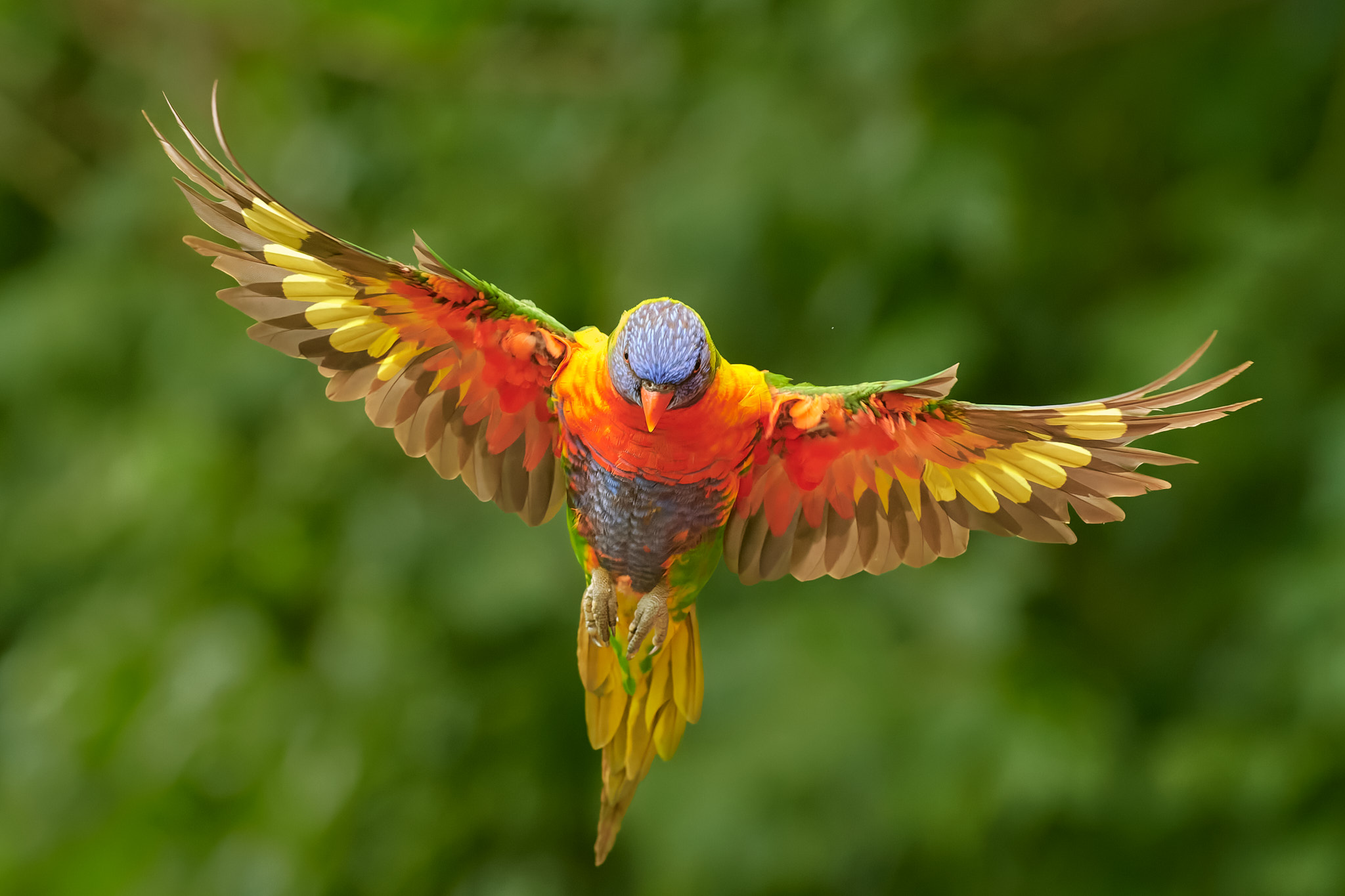The image captures a stunning and colorful bird mid-flight, with the perspective looking up at the bird as it soars towards the viewer. The bird's wings are fully spread, showcasing an intricate pattern and vibrant spectrum of colors. The underside of the wings and belly feature a beautiful muddle of yellow, red, and orange feathers, interspersed with brown edges. The bird's back and upper wings exhibit shades of green transitioning into red, orange, and light orange hues, eventually blending into yellow, brown, light brown, and beige tones. The head of the bird is adorned with blue feathers, an orange beak, and distinct black lines around the eyes and near the beak. There are also patches of blue and brown feathers around its face. The belly carries a prominent blue section topped with orange and yellow hues. The tail, visible from underneath, displays olive and yellow feathers. Surrounding the bird, the background is slightly blurred, revealing hints of green trees or plants, which emphasize the bird’s striking and vivid presence against the natural setting.